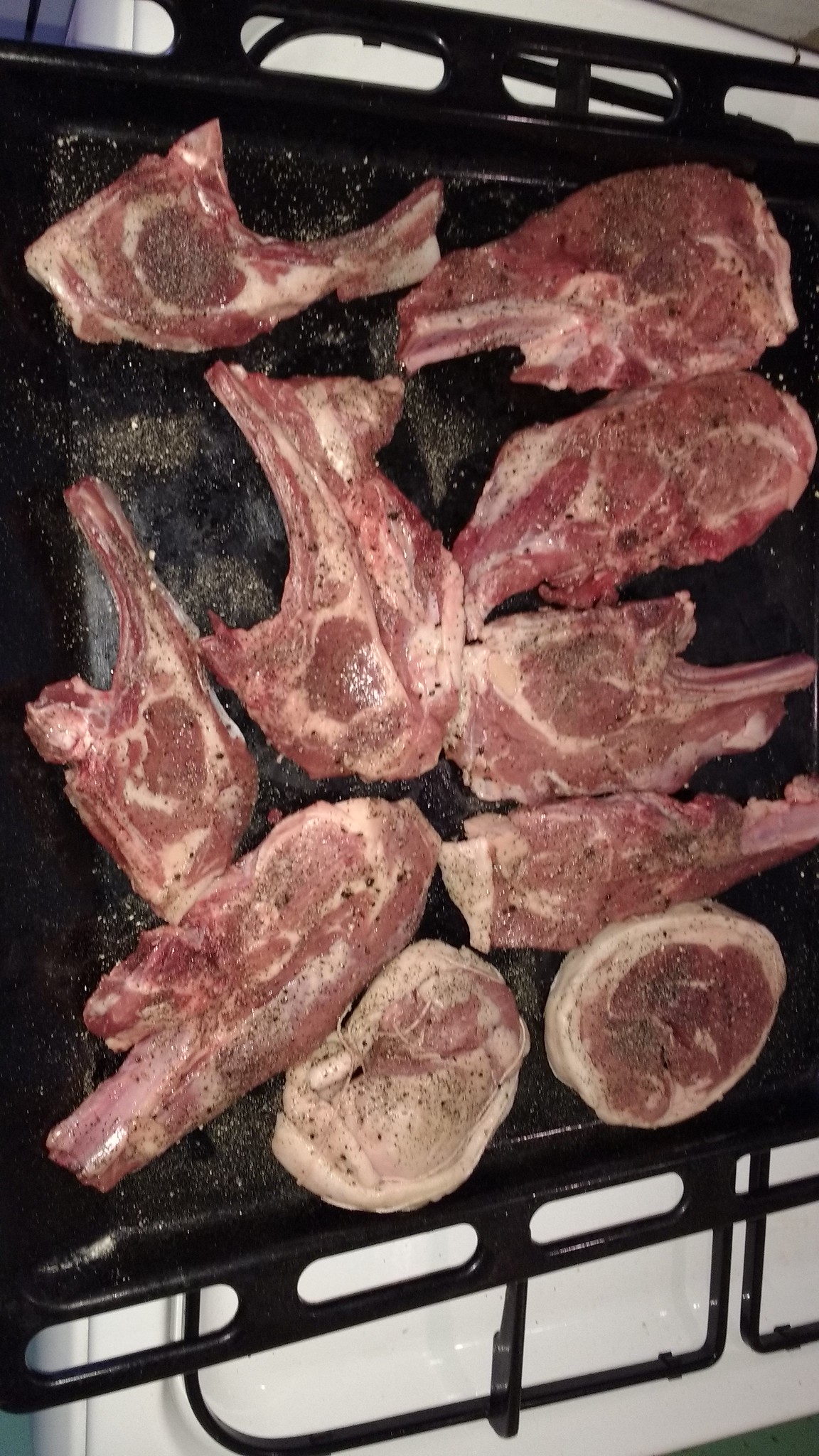The image showcases an upper view of a black ceramic-coated baking tray with white spots, sitting on a white, gas-burning stove in a kitchen. The tray holds multiple uncooked cuts of meat, including around eight steaks and two pork chops. The meat appears to be a blend of red and beige tones and is seasoned with crushed pepper and other spices, likely including salt. The pieces of meat display a mix of fat and muscle, with some portions being noticeably more tender and fatty than others. The tray features drip holes and hand slots, suggesting it is designed for easy handling and drainage. The stove beneath is not turned on, indicating that the meat is likely prepped and ready to be placed in the oven soon.